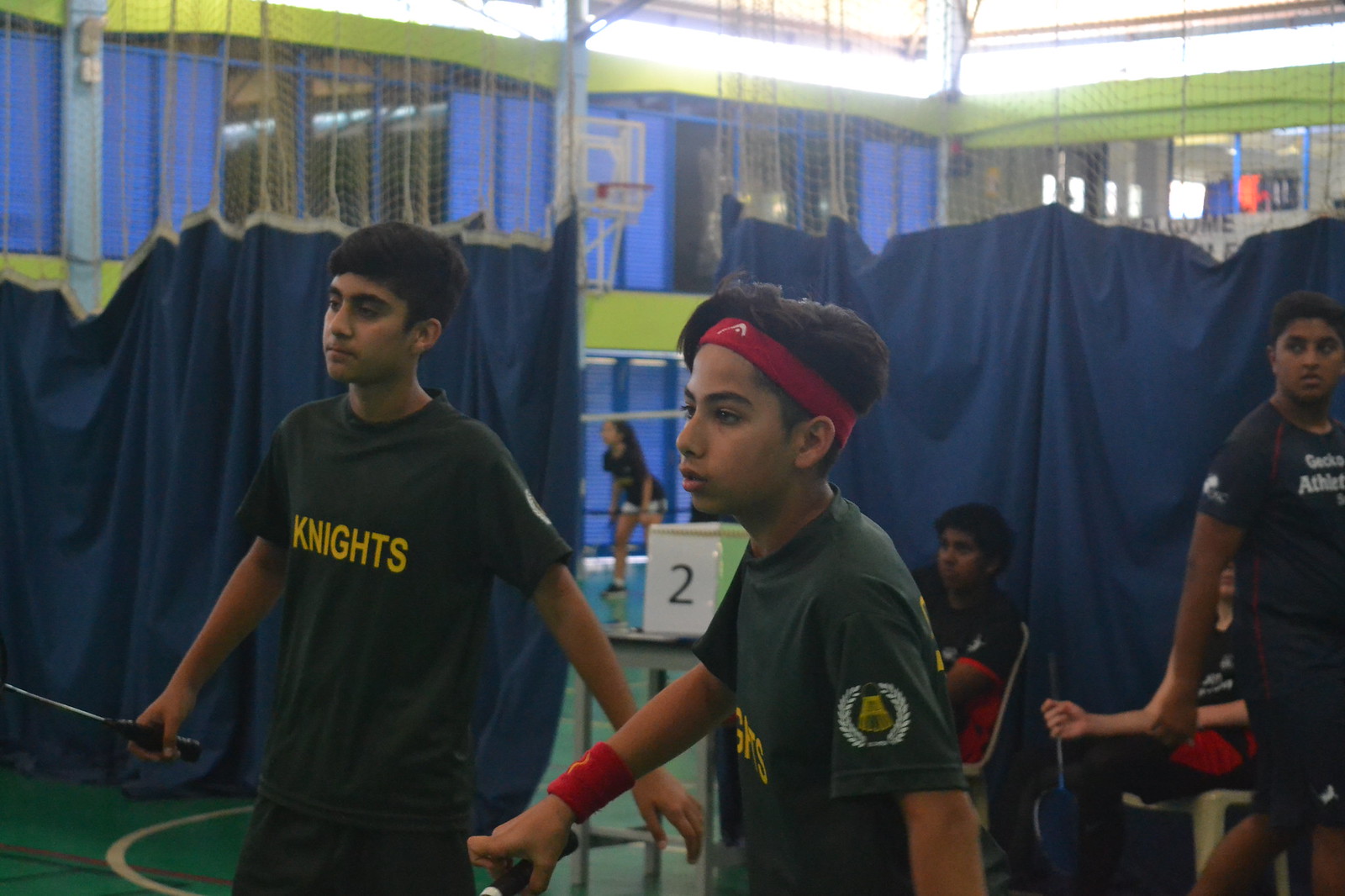This indoor photograph captures a group of boys engaged in a sporting activity within a school gymnasium. The setting is characterized by blue drapes with netting on top, acting as a divider across the middle of the gym floor. In the background, additional nets can be seen, along with a basketball hoop mounted on the wall. Two boys stand prominently in the foreground, each holding what appears to be a racket, though the netting of the rackets is not visible. Both boys have brown skin, short hair, and are dressed in short-sleeved, dark green shirts with the word "Knights" in yellow text on their chests. The boy on the right sports a red athletic headband and a matching wristband. Behind them, more boys dressed similarly are seated against the blue fabric barrier. A white card with a black number two is placed on a small table visible between the standing boys. Farther in the background, another group is engaged in volleyball, indicating a multi-sport environment in the gymnasium.